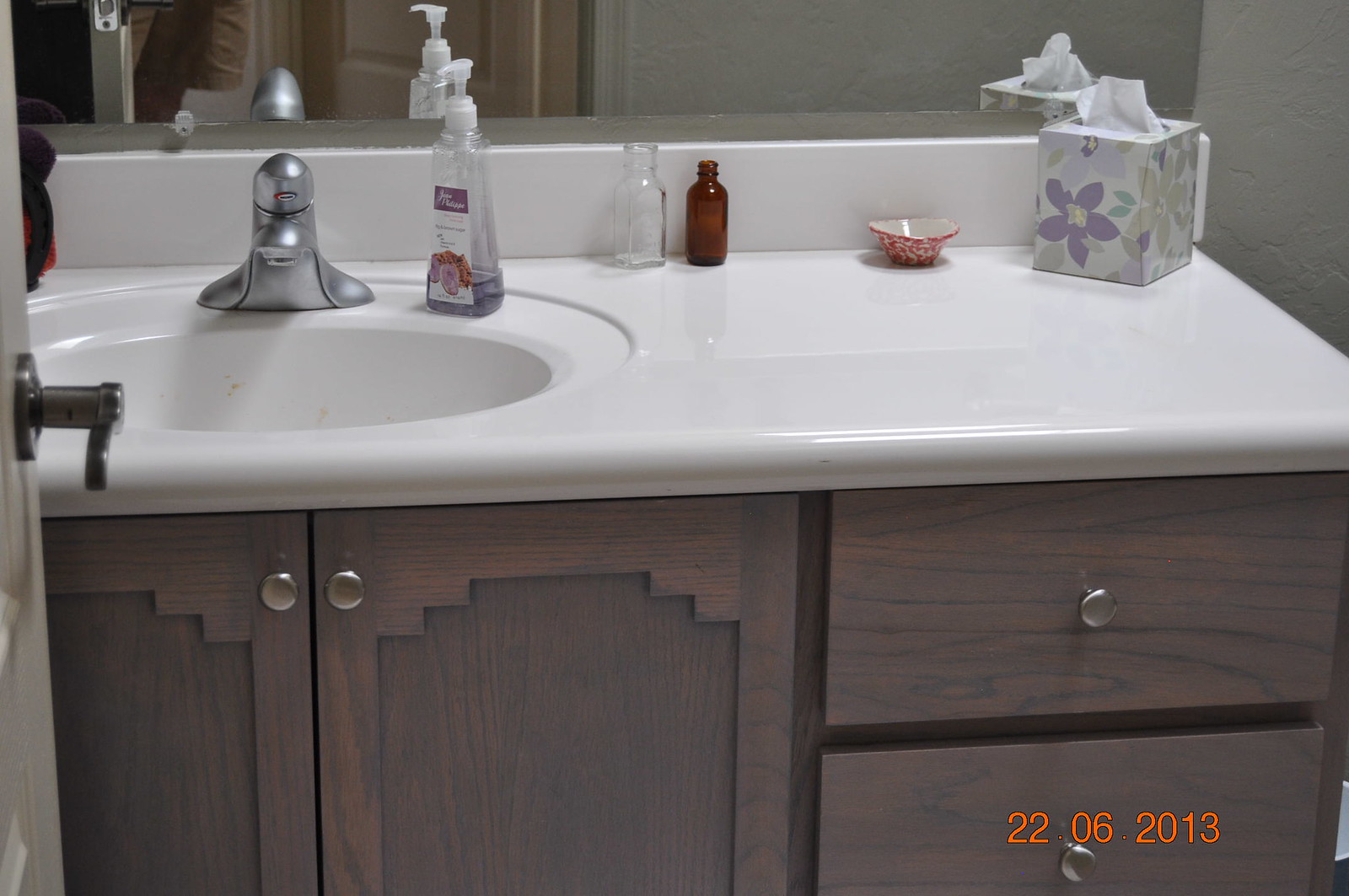Aimee stands next to a pristine white sink in this photo dated June 22, 2023. The countertop is adorned with a bottle of soap on the left, ensuring cleanliness, while the chrome faucet gleams under the light. To the right, a neatly placed tissue box adds a touch of practicality. The scene captures a moment of everyday simplicity and functionality.